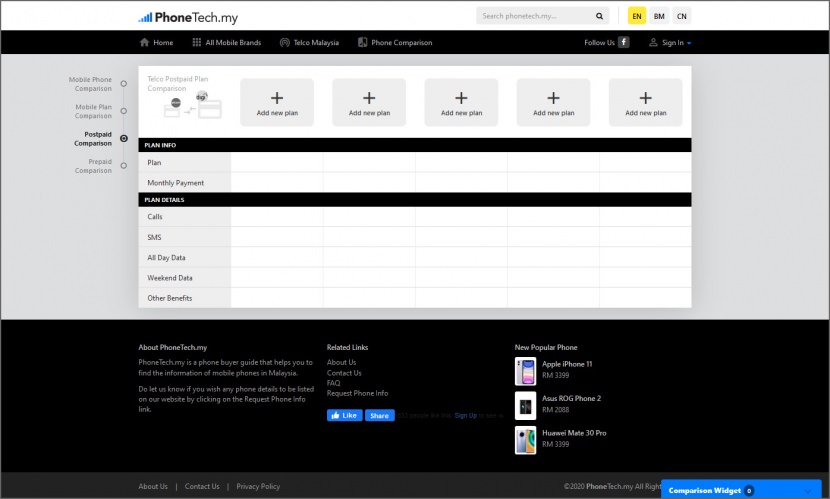This is a detailed screenshot from a page within the Phonetech.my website. The page header is located at the top left corner, featuring the Phonetech.my logo and name. Below the header, there are five horizontal bars, each shaded in progressively deeper shades of blue. 

On the top right, there is a gray search bar with an embedded magnifying glass icon. Adjacent to the search bar are three buttons labeled "EN," "BM," and "CN," which represent different language options. The "EN" button is highlighted in yellow, indicating that English is currently selected.

Beneath the language options, there is a navigation bar with links labeled "Home," "All Mobile Bands," "Phone Companion," and "Take Malaysia." To the far right of this navigation bar, there are links for "Facebook Follow Us" and "Sign In," both presented on a black background.

Below the navigation bar, a large gray box contains a smaller white box intended for adding personal plans. Within this section, the "Postpaid Companion" is chosen from the following four options: "Mobile Phone Companion," "Mobile Plan Companion," "Postpaid Companion," and "Prepaid Companion."

At the top of this section, there are five boxes featuring plus signs, each labeled "Add New Plan." Each plan has fields for entering the plan name, monthly payment, and additional details such as calls, SMS, all-day data, weekend data, and other benefits.

At the bottom of the page, there are related links for user engagement. These links include "About Us," "Contact Information," "FAQ," and "Request Phone Info." Additionally, there are images and names of three new phones displayed.